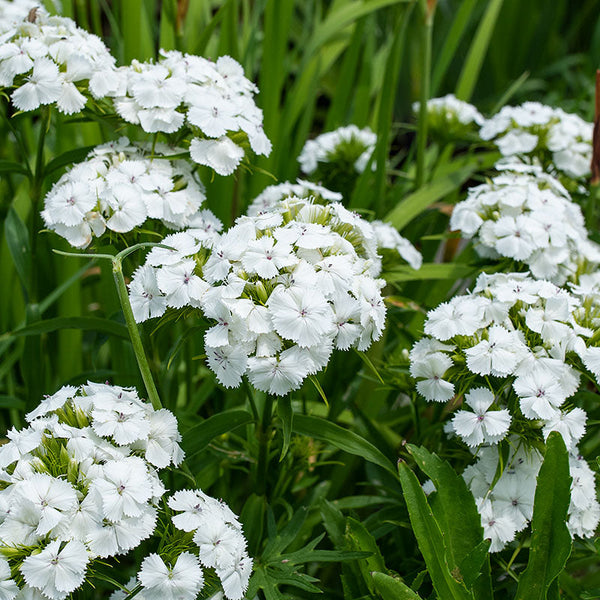This image captures a lush field of wildflowers interspersed with tall, unkempt green grasses, some of which show brown tips, indicating a natural and untamed setting. The field is dotted with delicate, clustered white flowers, each stem bearing approximately 15 to 20 petite blooms. These dainty flowers often feature a reddish dot at their centers, adding a touch of contrast to their predominantly white petals. The flower heads appear both full and partially depleted, suggesting a dynamic and natural scene. The flowers are scattered throughout the image, with the foreground in sharp focus and the right-hand side in a soft blur. The blurred background highlights the tall, slender leaves behind the blossoms. In the central part of the photograph, there is a prominent cluster of blooms, with the right side showing a vertical row of three flowers. A large bloom is partially visible at the lower left, while two smaller flowers peek out from behind the central cluster. The overall composition presents a picturesque and detailed portrayal of wildflowers in their natural habitat.